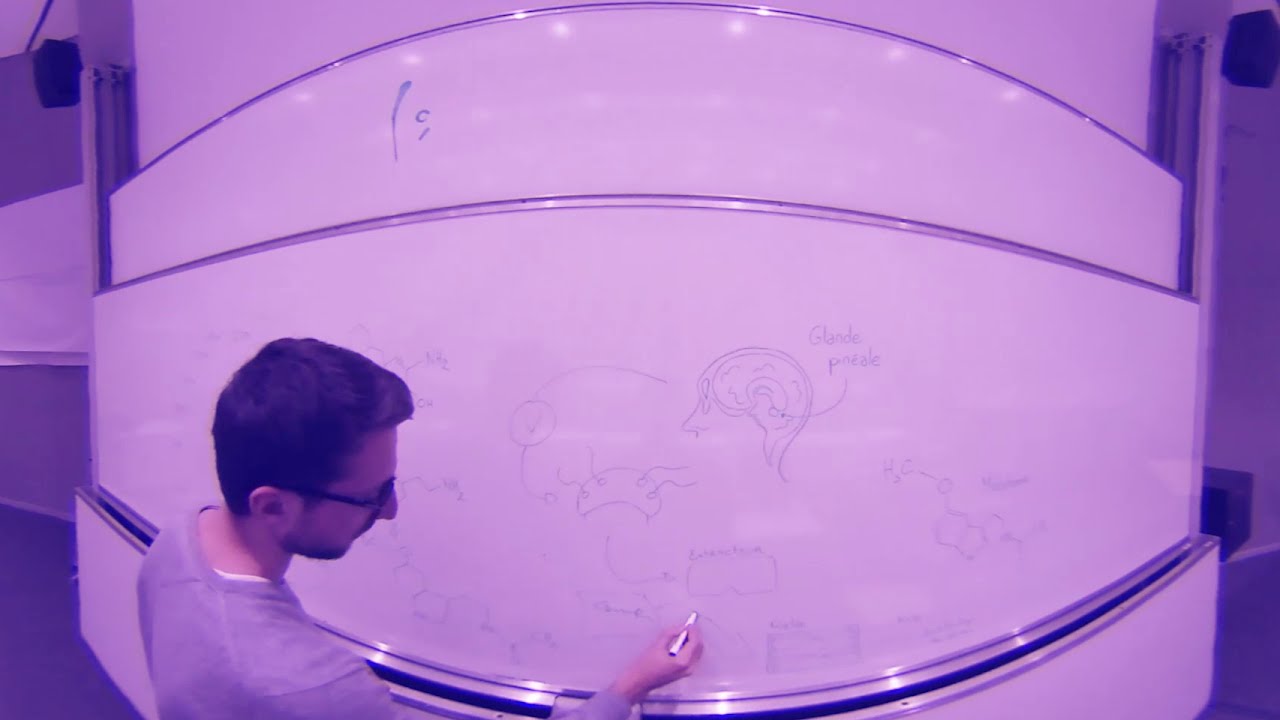In this detailed image, we observe a young male professor, likely in his early 30s, positioned in the bottom left corner of the scene. He is engaging with a dry erase board that dominates the center of the photo. The man has short brown hair and wears black plastic-rimmed glasses, a gray long-sleeve sweater, and a white t-shirt that peeks out from the collar. He appears to be drawing various detailed anatomical illustrations, including the top of a human skull, the brain inside it, and several accompanying diagrams such as a curved disc with four holes. He holds a marker in one hand, actively working on the board.

The background suggests an indoor, classroom setting, but the exact time of day is indeterminate. The whiteboard is covered with multiple depictions, including some possibly related to chemicals, and text written in a language other than English, with phrases such as "glande finale" pointing to parts of the brain. The entire image carries a purplish tint that affects the visible color palette, making it dominated by shades of dark purple, light purple, black, silver, white, and gray. The image appears slightly warped at the edges due to the wide-angle shot, emphasizing the central focus on the professor and his intricate drawings on the board.